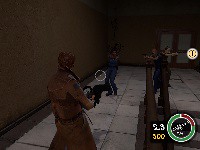The screenshot appears to be from an early 2000s video game, possibly from a game like "Postal." It features retro-style graphics and is predominantly dark, making it hard to discern details. The perspective is from a third-person viewpoint of a man with brown hair, wearing a brown trench coat, and seemingly wielding a weapon, possibly a cat based on the "Postal" series' notoriety. He stands on a notably bright, white tiled floor. In the center of the screen is a white circle with a dot, indicating the weapon's aim. Opposite him, three figures also hold weapons pointed in his direction. The background shows brown walls and a couple of doors with windows. The bottom right corner of the image displays a player stats interface, featuring a hollow circle with a green bar that transitions to red, likely representing health or wellness, and numerical indicators such as the number 23 in white and 300 in yellow, probably related to the player's ammunition count.